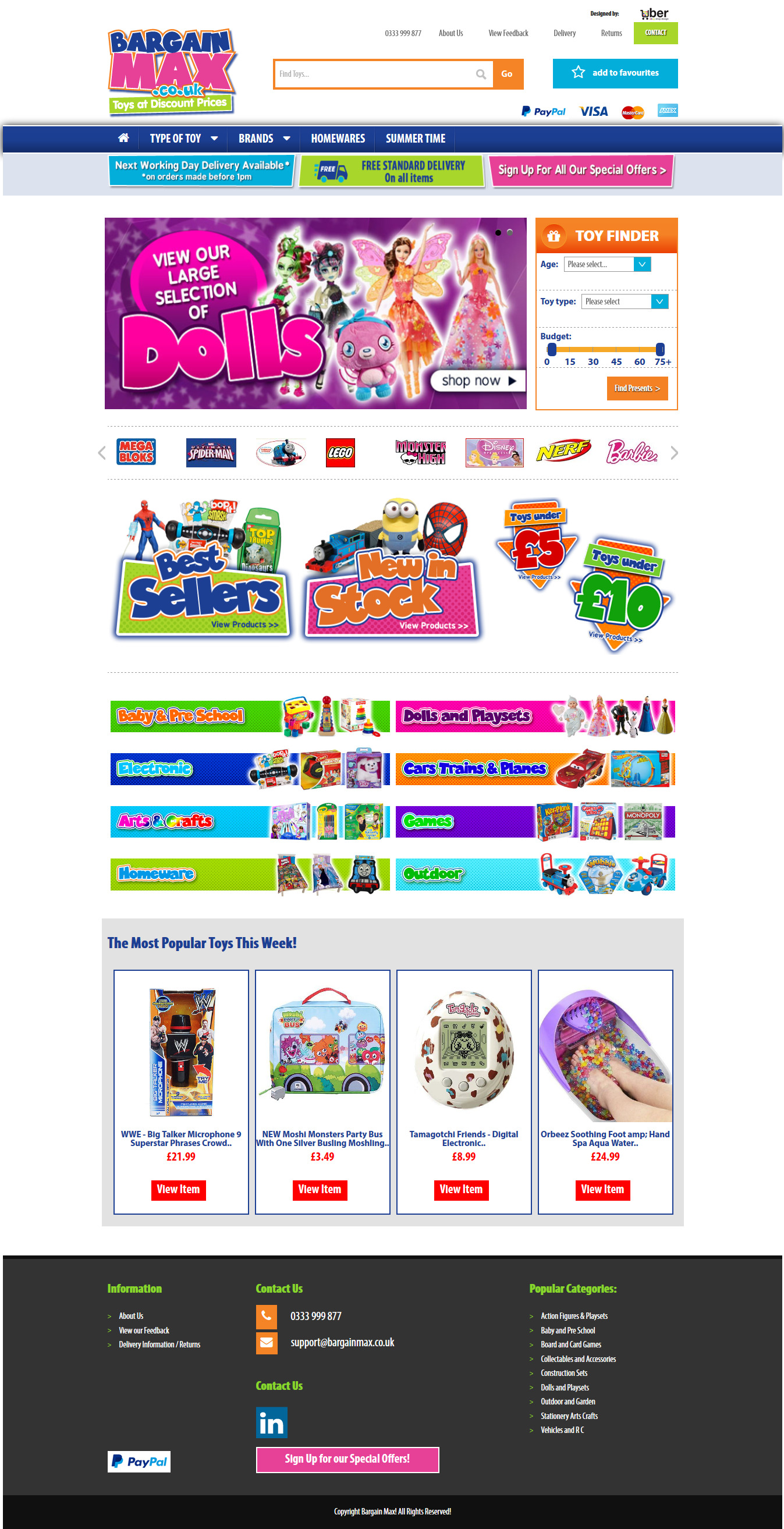This image is a screenshot from a website with a white background. At the very top of the screenshot, the header on the upper left-hand side displays the brand name “Bargain Max.” The word "Bargain" is written in a navy blue font, while "Max" is in a pink font. Beneath the header is a narrow navy blue navigational menu with white text that is unfortunately too small to read clearly.

Below the navigational menu, there is a prominent graphic that spans almost two-thirds of the width of the image, featuring shades of purple in the background. This graphic invites viewers to “view our large selection of dolls,” with the word "Dolls" highlighted in a very large pink font. To the right of this text are illustrations of various dolls. The doll in the far right corner of the image appears to be a Barbie doll dressed in a long antebellum-style evening gown. Next to that, there is another doll, likely a Disney character reminiscent of Tinkerbell, complete with wings.

Further down, the website is divided into three categories against a white background. The first category, on the left, is titled "Bestsellers," written in blue font within a green rectangle. The middle category reads "New in Stock," using an orange font against a pink background. Underneath these sections, several additional categories are displayed side by side in two rows, with oblong shapes of different colors highlighting each category. Inside these shapes are small illustrations representing various types of toys, suggesting a diverse selection available for browsing.

This detailed description captures the visual elements and layout of the website screenshot, giving a comprehensive overview of what is presented in the image.